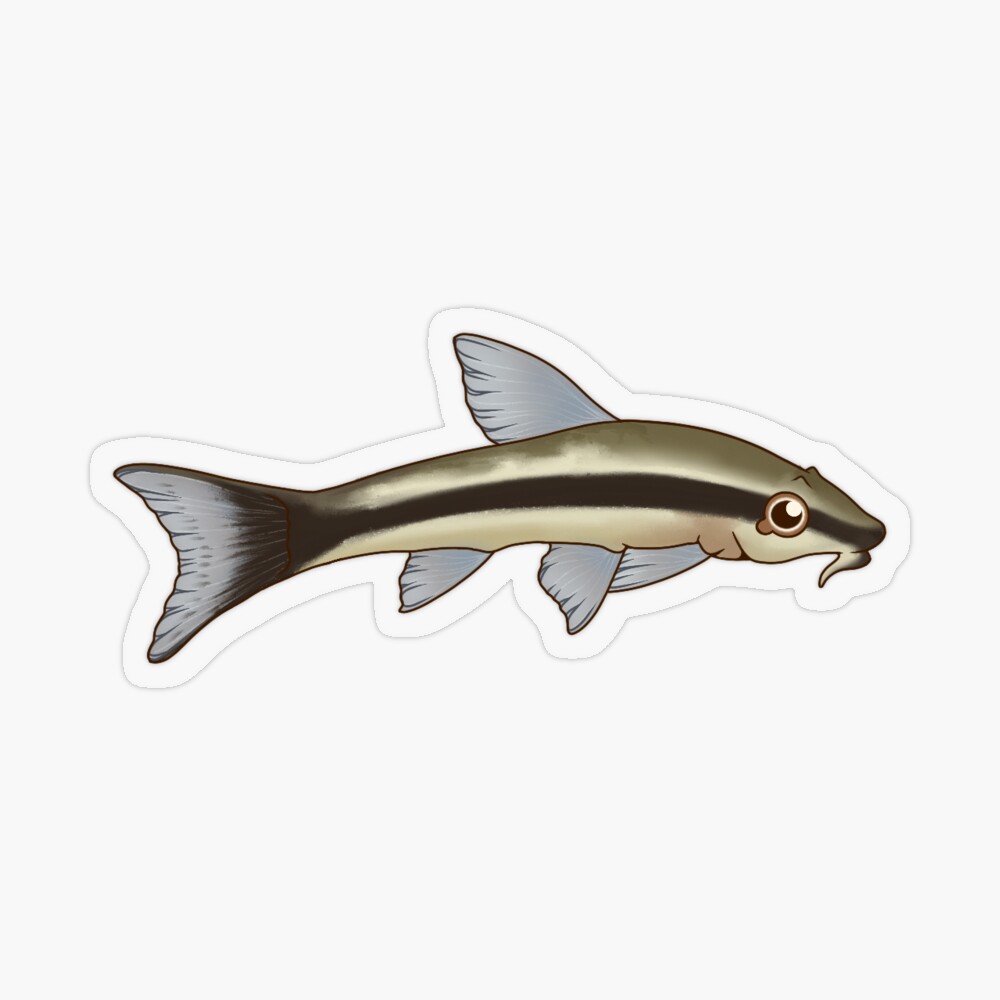This image features a small, long, cartoonish fish designed as a decal or sticker, prominently placed in the center of a white background within a wide vertical rectangular frame. The fish faces to the right and has a distinct white outline, complemented by a subtle gray drop shadow that accentuates its sticker-like design.

The fish's body showcases a dark stripe running longitudinally from its nose to its tail, flanked on either side by lighter colors. The upper part of the fish is a mix of dark gray with subtle white streaks, while the lower body transitions to a white or off-white, eggshell hue. The top spine area of the fish has a darker brown shade, and the belly portion appears beige.

The fins, colored in various shades of gray to light blue, are arranged with three on the bottom—one near the tail, one in the middle, and one close to the gills—along with one large fin on top and a tail fin. The fish has a prominent, round eye characterized by a large black pupil and a small white circle indicating a light glint.

Under the fish's mouth, there's a distinctive protruding feature that resembles a short whisker or a half tooth, similar to the feelers on a catfish but shorter and stouter.

The fish's overall design, with its detailed and vibrant color contrasts, rounded eye, and unique protrusion under the mouth, gives it an engaging, cartoon-like appearance, perfect for a sticker.